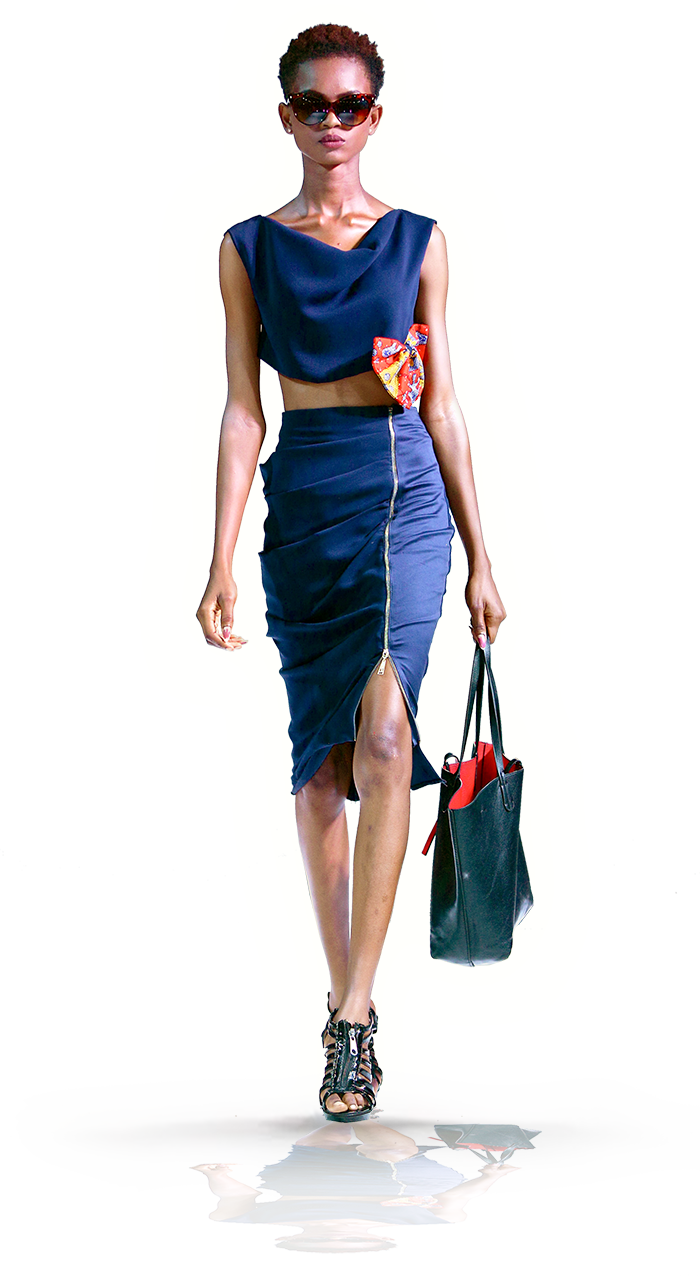A photograph displays a tall, lean, light-skinned African-American woman with short dark hair, exuding the aura of a model. She stands confidently in front of the camera, revealing a strong yet elegant posture accentuated by prominent collarbones and slender limbs. Her striking look is complemented by large sunglasses obscuring her eyes, adding an air of mystery. She is clad in a chic blue outfit consisting of a cropped top and a matching skirt with a distinctive gold zipper running from her waist to her knee, partially open to reveal one knee. Cinched at the waist is a belt adorned with a colorful bow featuring shades of red, blue, yellow, and white. As for her accessories, she carries a large black leather handbag with a vivid red lining and sports stylish black high-heeled shoes, each embellished with a zipper, showcasing her white-painted toenails. The overall appearance is polished, poised, and fashion-forward, ideal for a runway or fashion editorial. For more information, visit www.FEMA.gov.